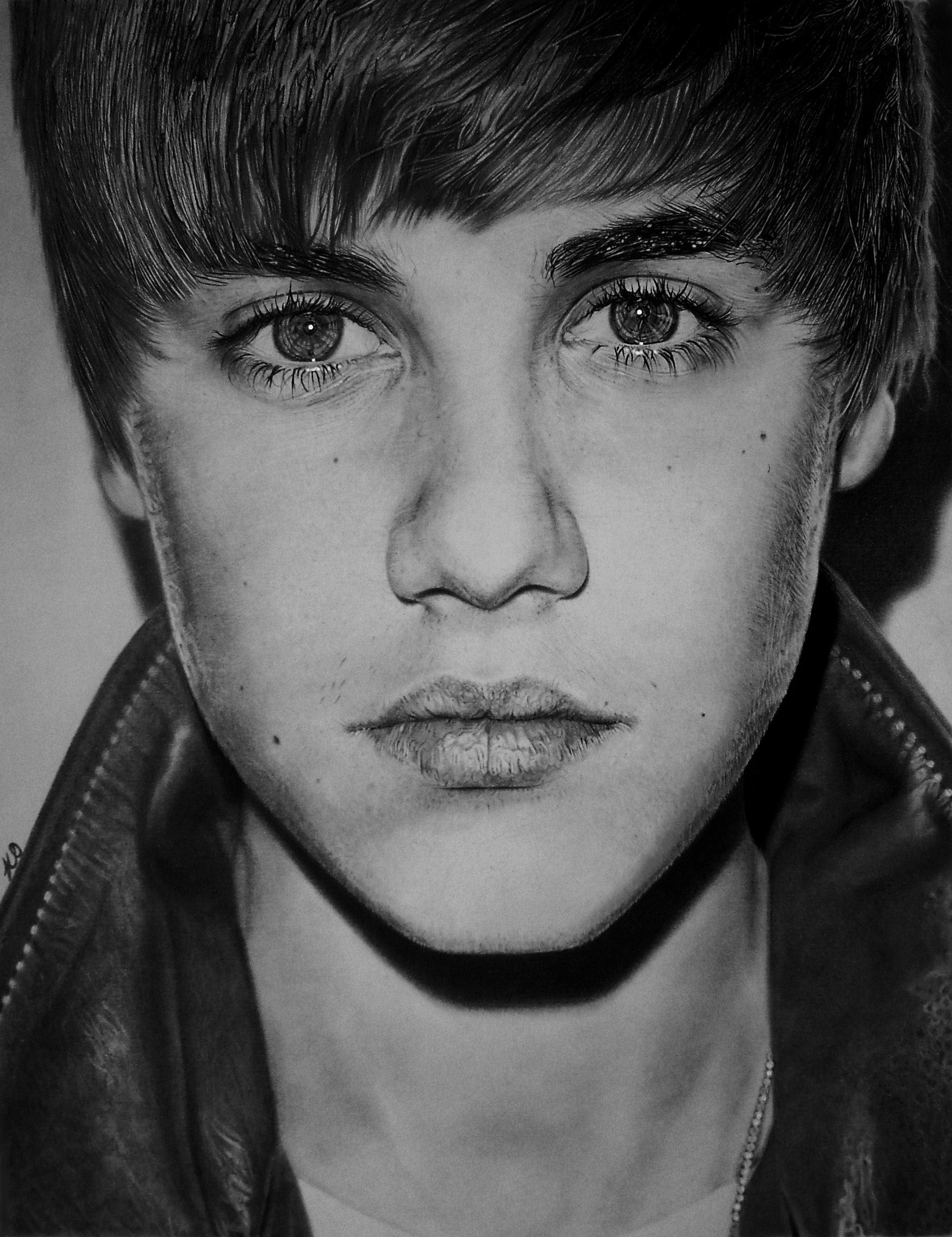The image is a vertically aligned, extreme close-up, black and white portrait of a young male celebrity, whose identity isn't specified though he vaguely resembles Justin Bieber. The photograph is highly zoomed in, with the face filling most of the frame and cut off at the base of the neck. The young man has dark eyes, long eyelashes, dark eyebrows, and long bangs that are combed down over his forehead and sides, partially covering his dark hair. His mouth is closed, with lips that appear glossy. He wears a black leather jacket with a high collar turned up, detailed with white stitching, over a white t-shirt that's mostly out of frame. Around his neck, he sports a thin metallic chain necklace. The background is a solid white, and the proximity of the figure to the backdrop is emphasized by the shadows cast behind him. His expression is stern and serious, and although the side of his face is somewhat shaded, it is clear he isn’t sporting any facial hair.